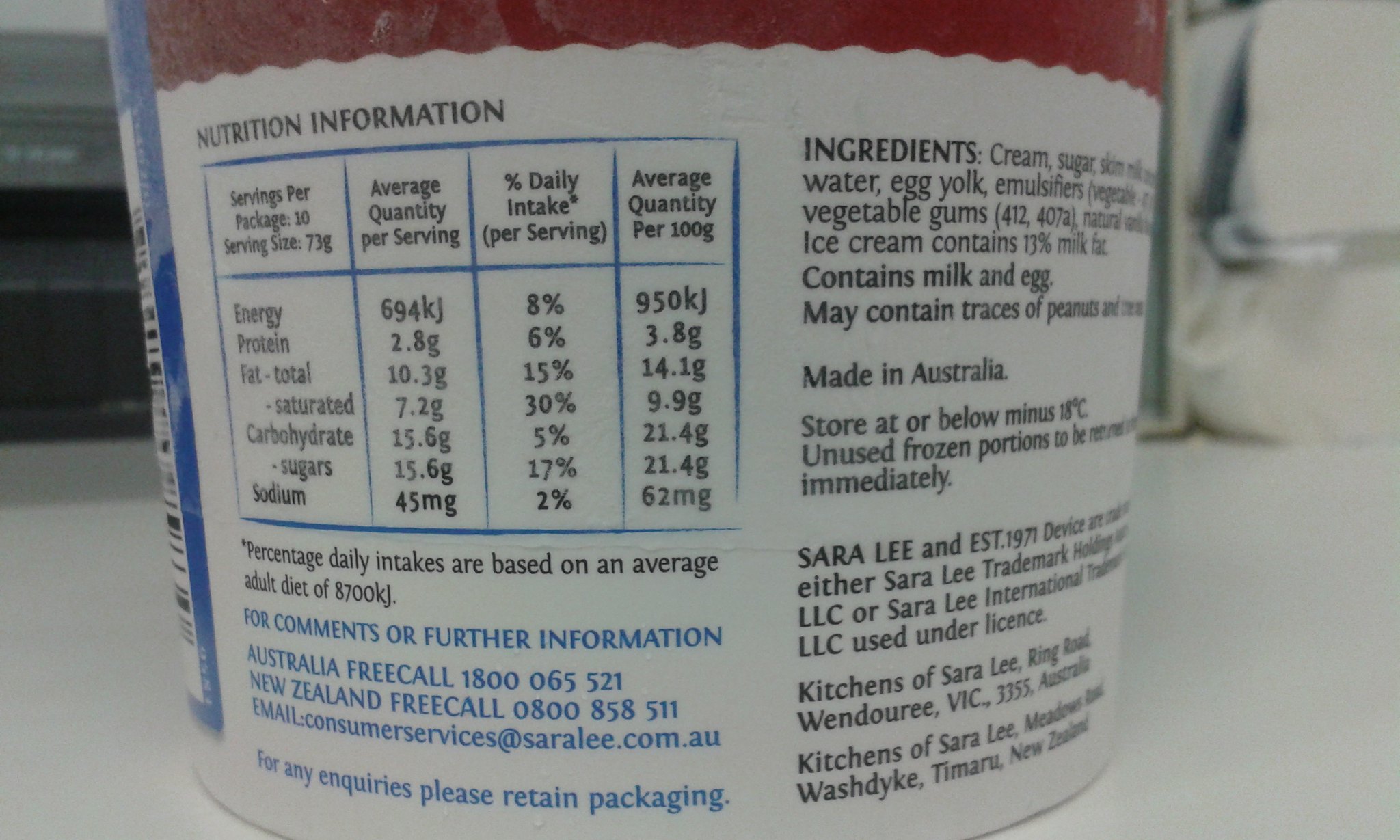**Detailed Caption:**

The image features a nutritional information label on the back of a classic round plastic container, possibly an ice cream carton. The top of the container is cut off just below the lid, and the bottom is slightly obscured. The container is placed on a white surface, with some white objects in the upper right corner and a device that might be a VCR in the left corner.

The nutrition information is prominently displayed, outlined in a large rectangular box with blue lines. The label details that the container holds 10 servings, with each serving size being 73 grams. It breaks down the average quantity per serving, percentage daily intake, and average quantity per 100 grams for various nutrients, including energy, protein, fat, saturated fat, carbohydrate, sugar, and sodium. Additionally, it notes that the percentage daily intakes are based on an average adult diet of 8,700 kilojoules.

For further comments or information, two contact numbers are provided: Australia free call with a phone number, and New Zealand free call with a phone number. There's also an email address: consumer.services@saralee.com.au, indicating the brand is Sarah Lee.

On the right side of the label are the ingredients: cream, sugar, skim milk, water, egg yolk, emulsifiers, vegetable gums, and natural flavoring. The product is identified as ice cream, containing 13% milk fat. Allergen information notes that it contains milk and egg and may contain traces of peanuts and tree nuts.

The product is made in Australia and should be stored at or below -18°C, with unused portions to be returned to the freezer immediately. The label also mentions "Sarah Lee, established 1971" with trademark warnings and an address for Australia and New Zealand.

Much of the label is white with blue lettering and accents. A blue rectangular stripe is visible on the left-hand side of the container, and a red scalloped border decorates the top edge.